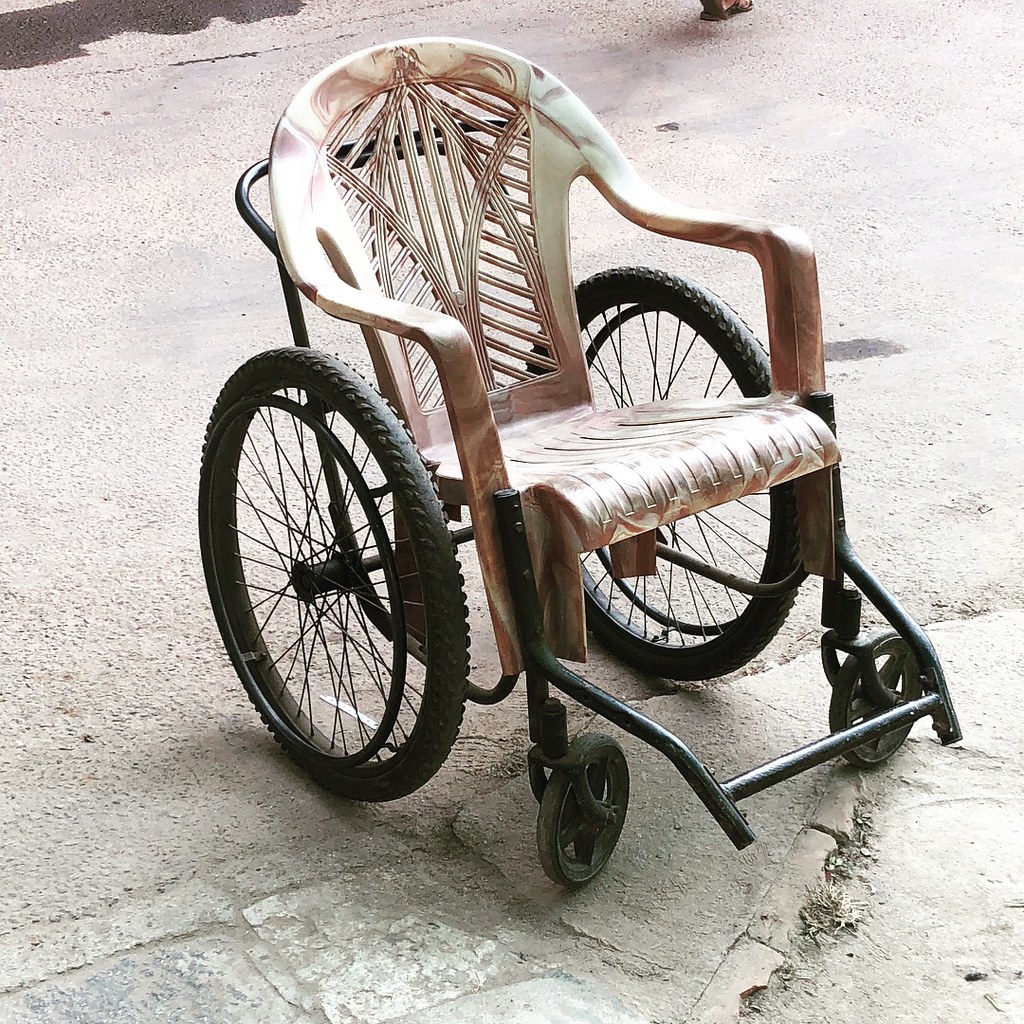The photograph depicts a makeshift wheelchair, distinctly cobbled together from unconventional materials. The seating area features a plastic chair, cream and peach-colored with brown patterns, whose legs were shortened and securely attached to the wheelchair's frame. The chair includes armrests and a semi-circular back with openings typical of plastic garden furniture. The wheelchair has two large black wheels at the rear and two smaller wheels at the front for direction and support. The metal frame of the original wheelchair is black, providing a sturdy base for the makeshift seat. The setup is placed on a concrete or stone ground, giving the scene an industrial and rugged feel. In the upper part of the image, the foot of a person is faintly visible, adding a subtle human element to the scene.